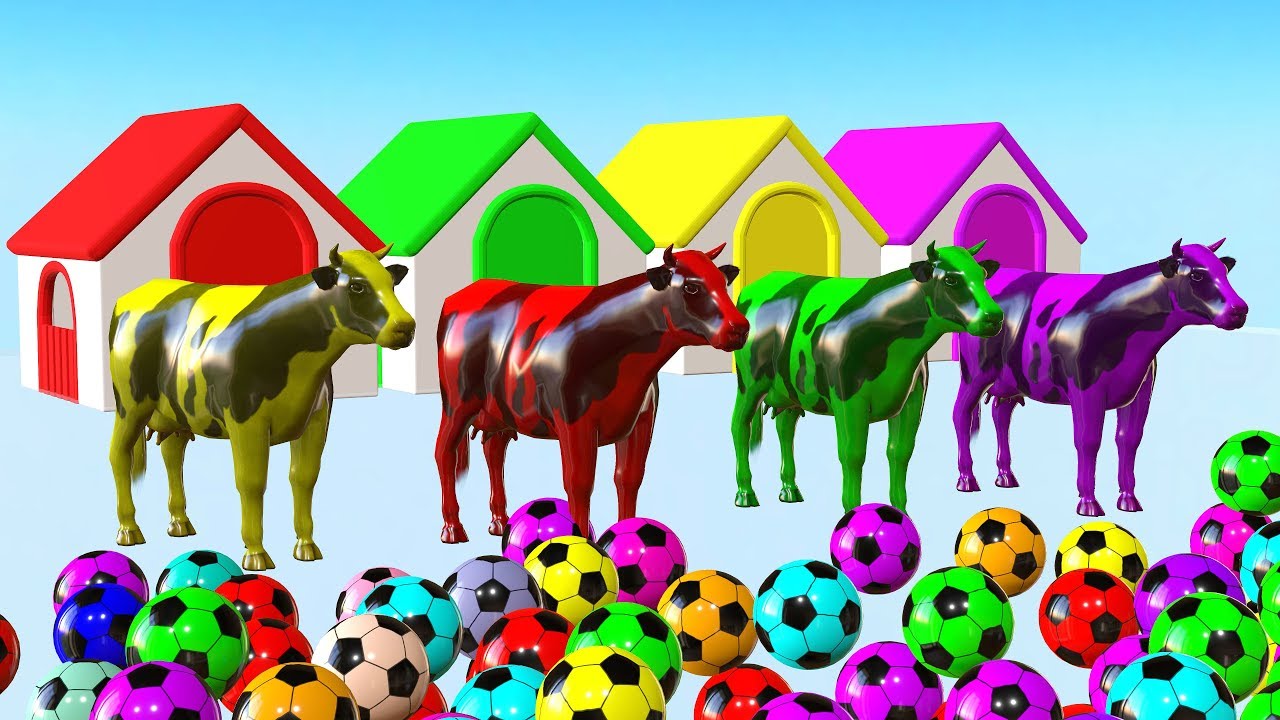The image is a detailed graphic art or illustration showcasing a vibrant scene featuring toys against a dynamic background. Four houses or barns, each with a triangular roof and an arched doorway topped by an arched window, are lined up in the middle of the image. They display a gradient from a blue background at the top to a whiter bottom section. Each house shares a uniform structure but is distinctively colored: the first house is red, the second is lime green, the third is bright yellow, and the fourth is fuchsia purple.

In front of each house stands a colored cow figurine. Corresponding to the houses, the first cow is black and yellow, the second is black and red, the third is black and green, and the fourth is black and purple. These cow figurines appear to be plastic or computer-rendered rather than hand-drawn.

Scattered in the foreground are numerous soccer balls, rendered in various colors including purple, blue, turquoise, lime green, light orange, red, and various shades of purple. The whole scene is bathed in a playful and whimsical color scheme, creating an engaging and lively tableau.